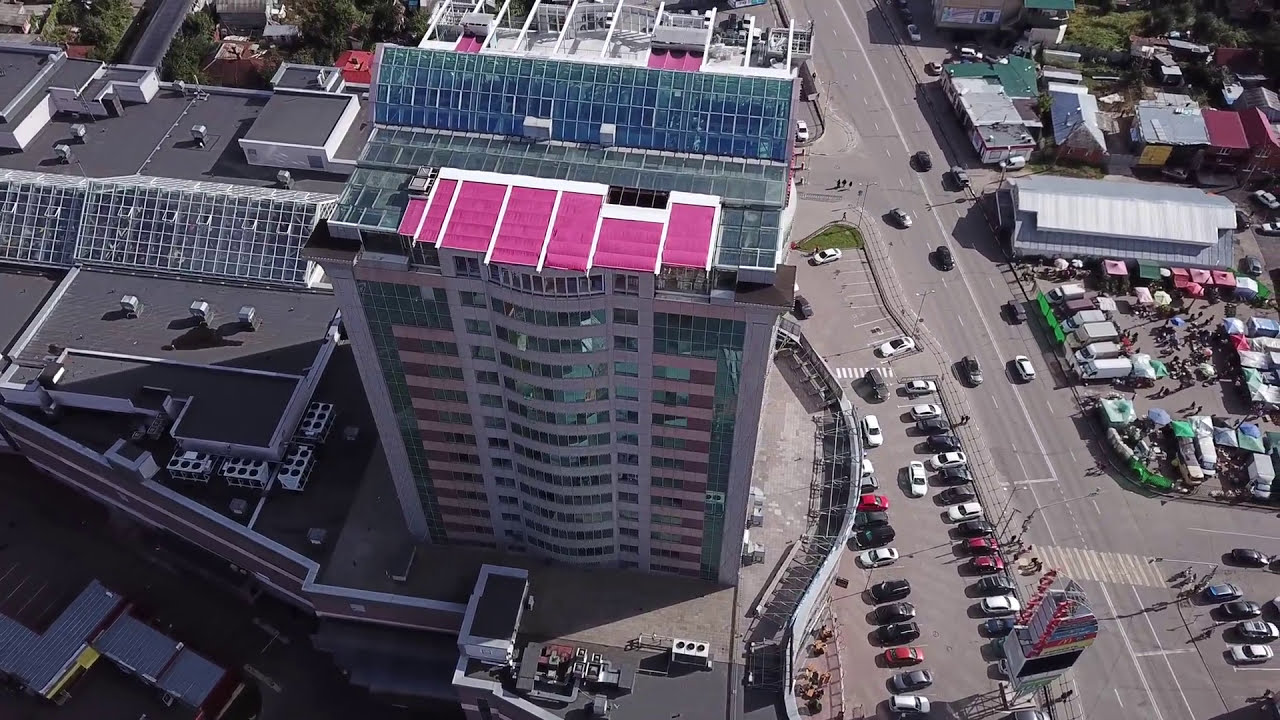This color photograph is an aerial view, likely taken from a drone or a helicopter, capturing a bustling urban scene on a bright, sunny day. At the center of the image stands a tall building with a strikingly unique roof, composed entirely of angled glass panels, interspersed with pink awnings that cover parts of the glass surface. The building also features numerous square windows along its facade, with blue panels adding to its distinctive appearance.

Below, the street scene reveals a busy environment with a multitude of black and white cars parked in neat rows beside the building. The main road runs between this central building and another bustling area on the right-hand side, where a lively market is in full swing. The market area is marked by a sea of colorful umbrellas, tents, and small trucks, with clusters of people navigating the vibrant space. Surrounding this scene are various other buildings, characterized primarily by their gray rooftops.

Overall, the image offers a detailed snapshot of urban life from a bird’s-eye perspective, highlighting both architectural details and the dynamic street activity below.